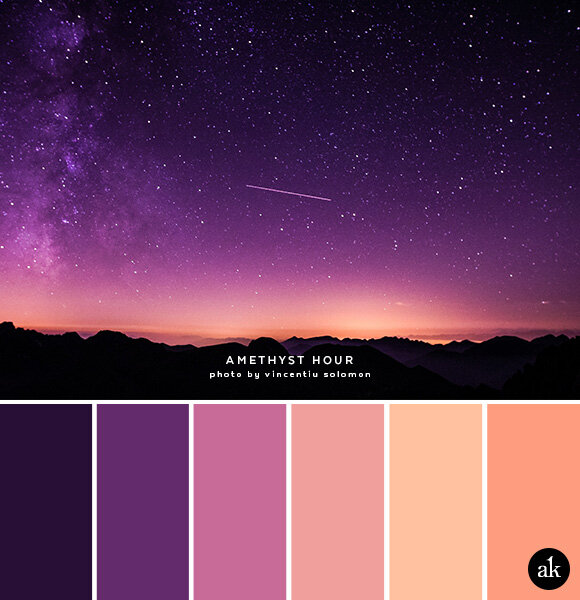The image titled "Amethyst Hour" by Vincentiu Solomon features a stunning photograph of the night sky, colorized in shades of purple with a gradient transitioning to a salmon-pink glow near the horizon. The sky is dotted with numerous white stars, and a faint white streak suggests a falling star. On the left, the gasses of a galaxy are faintly visible, enhancing the celestial scene. Below the sky, the rugged silhouette of black mountains adds contrast. 

The upper section of the image, dominated by this nighttime landscape, bears the photo’s title and photographer’s name in white text. The lower section of the image contains six solid color swatches extracted from the photograph. These swatches, from left to right, include indigo, violet, mauve pink, peach, a vibrant orange, and a deeper orange. In the bottom right corner, a black circle with the white lowercase letters "ak" in a serif font adds a subtle signature element to the composition.